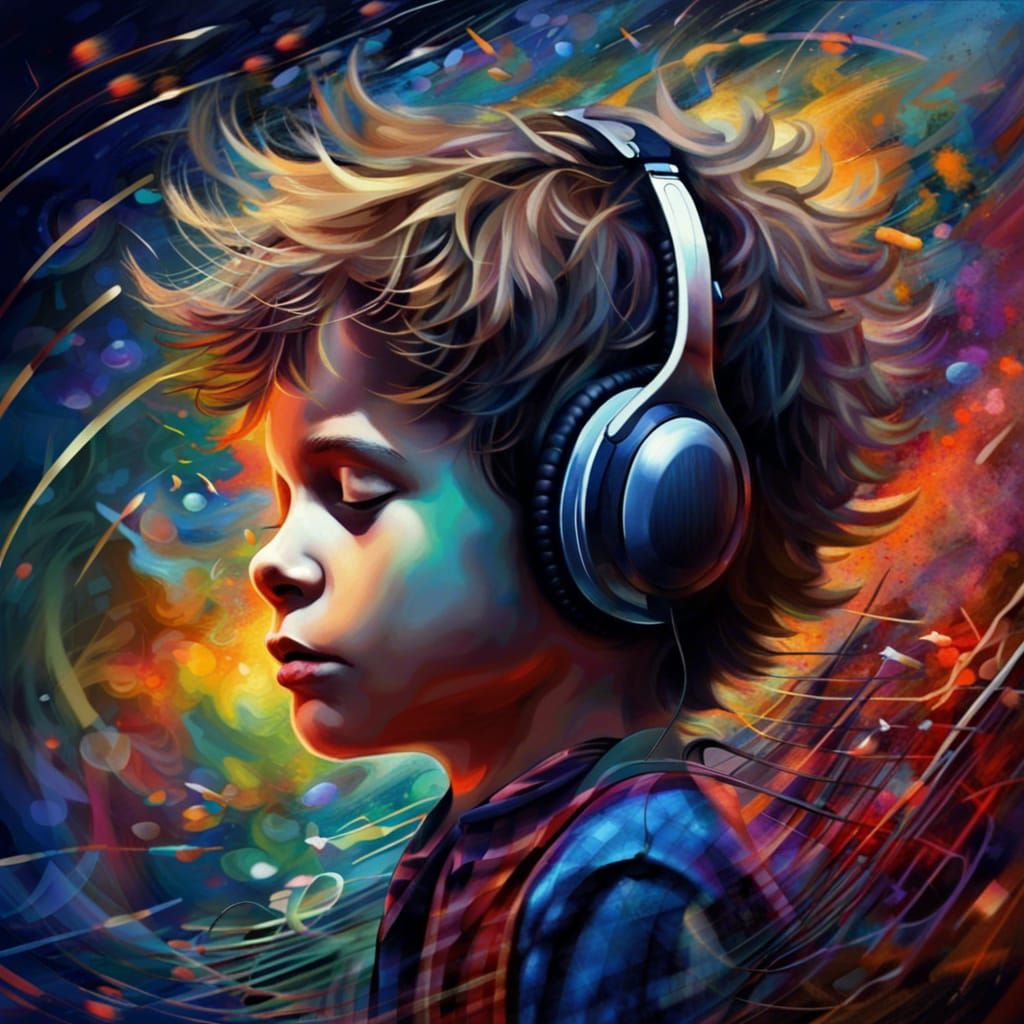This artwork is a vibrant and colorful drawing, rich in abstract swirls and strokes that fill the background with an array of colors, including red, orange, yellow, green, blue, and purple, interspersed with some black and white. The central figure is a young boy, around 8 or 9 years old, depicted in profile facing left. He has fair skin and neck-length, curly brown hair with a slightly messy, almost anime-inspired look. His eyes are closed, suggesting he is deeply absorbed in the music emanating from the gray and black over-the-ear headphones he is wearing. The boy is dressed in a blue shirt overlaid with a red vest or striped shirt, giving a layered outfit appearance. The background features dynamic swirls, primarily yellow behind his head, transitioning to darker blue and green towards the upper left, and warmer reddish-orange hues in the lower right, enhancing the overall sense of movement and emotion in the piece.